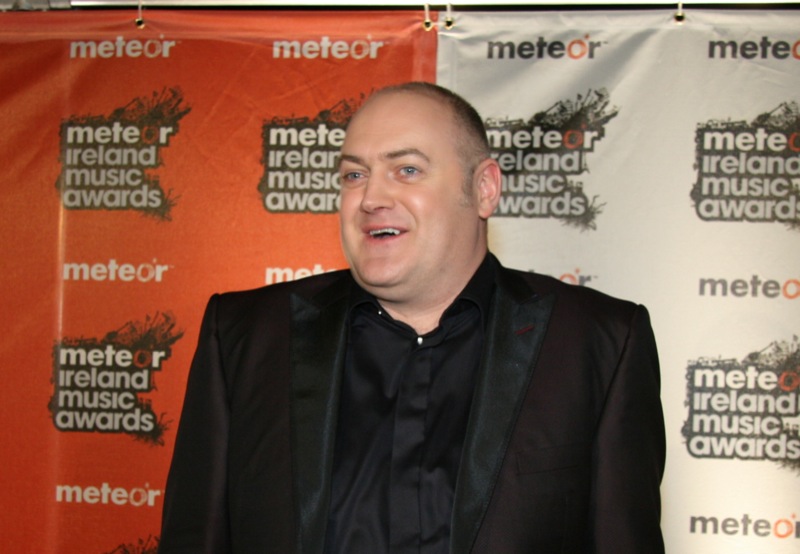This photograph captures a smiling, slightly overweight white male with a shaved head attending the Meteor Ireland Music Awards event. He is posed in the foreground wearing a black sport coat over a black dress shirt. The man seems to be caught mid-expression, with his mouth slightly open as if between smiles. The background is dominated by a large, split-color banner displaying the name of the event. The banner is divided vertically, with the left half in orange and the right half in white, and it features the text "Meteor Ireland Music Awards" in white font with a black outline. The banner spans the entire background, providing a clear and festive context for the event. The man appears in good spirits, embodying the celebratory atmosphere of the occasion.